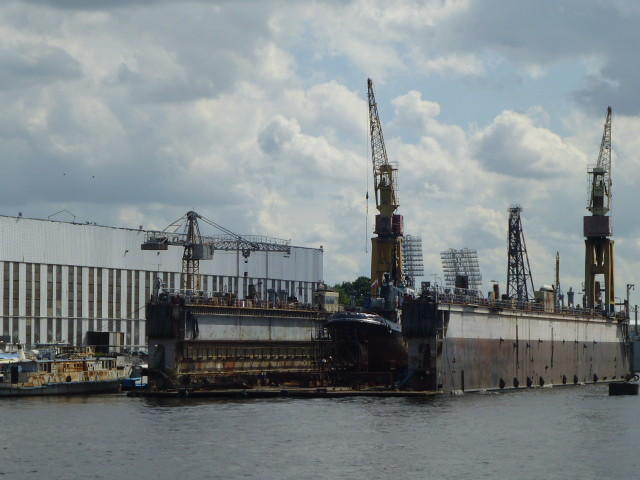The image captures a bustling shipyard set against the backdrop of a cloudy, overcast sky. Dominating the background is a large, white warehouse-like building with numerous rows of windows. The forefront of the image showcases a dock, where a ship is visible, though only partially—just the lip can be seen, elevated by machines for what appears to be repairs. This shipyard scene is filled with industrial activity, evidenced by the presence of multiple cranes, particularly one on the right-hand side and another on the left-hand side of the picture. The dock itself is flanked by other vessels, including a notably old and rusted boat situated on the left. The overall lighting is somewhat dim due to the cloud cover, casting a subdued light over the entire shipyard, and below the dock, the calm waters reflect the industrial landscape above.